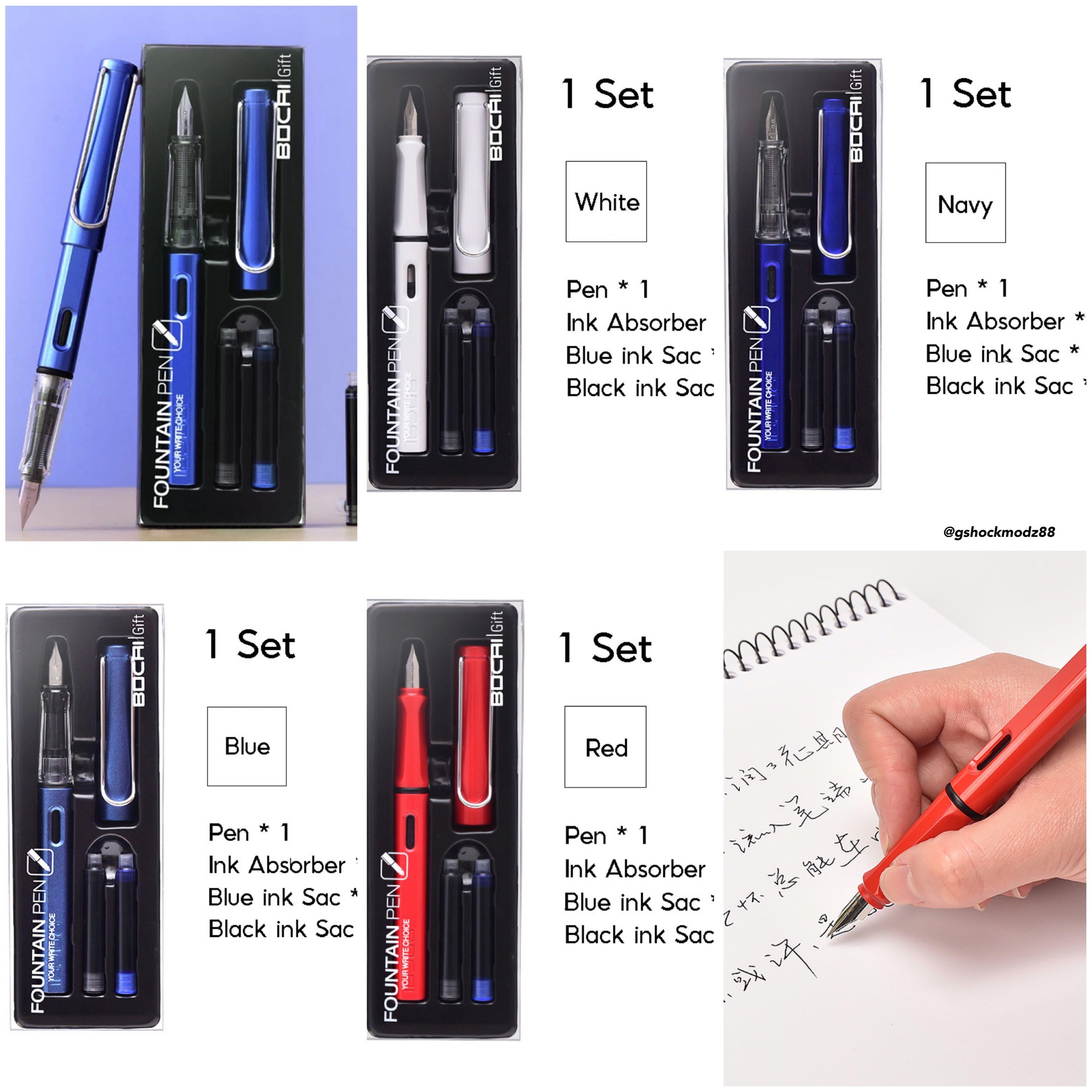The image features a detailed advertisement for a series of fountain pens displayed against a white background. The advertisement showcases five sets of pens, each housed in a vertically oriented rectangular section within a black display case, mimicking what you might see in a store. Each set contains a different colored pen: three are blue, one is white, and one is red. Every pen set includes a pen with blue, black, or navy ink options, an ink absorber, and blue and black ink sacks. The packaging prominently reads "White Ink" and "Fountain Pen" in white text, while a product description in black text details the contents of each set. In the bottom right corner of the image, there’s a picture depicting a white hand using a red pen to write on white paper with black ink. This section also includes partially legible text and the notation "© G-Shock Mods 88."